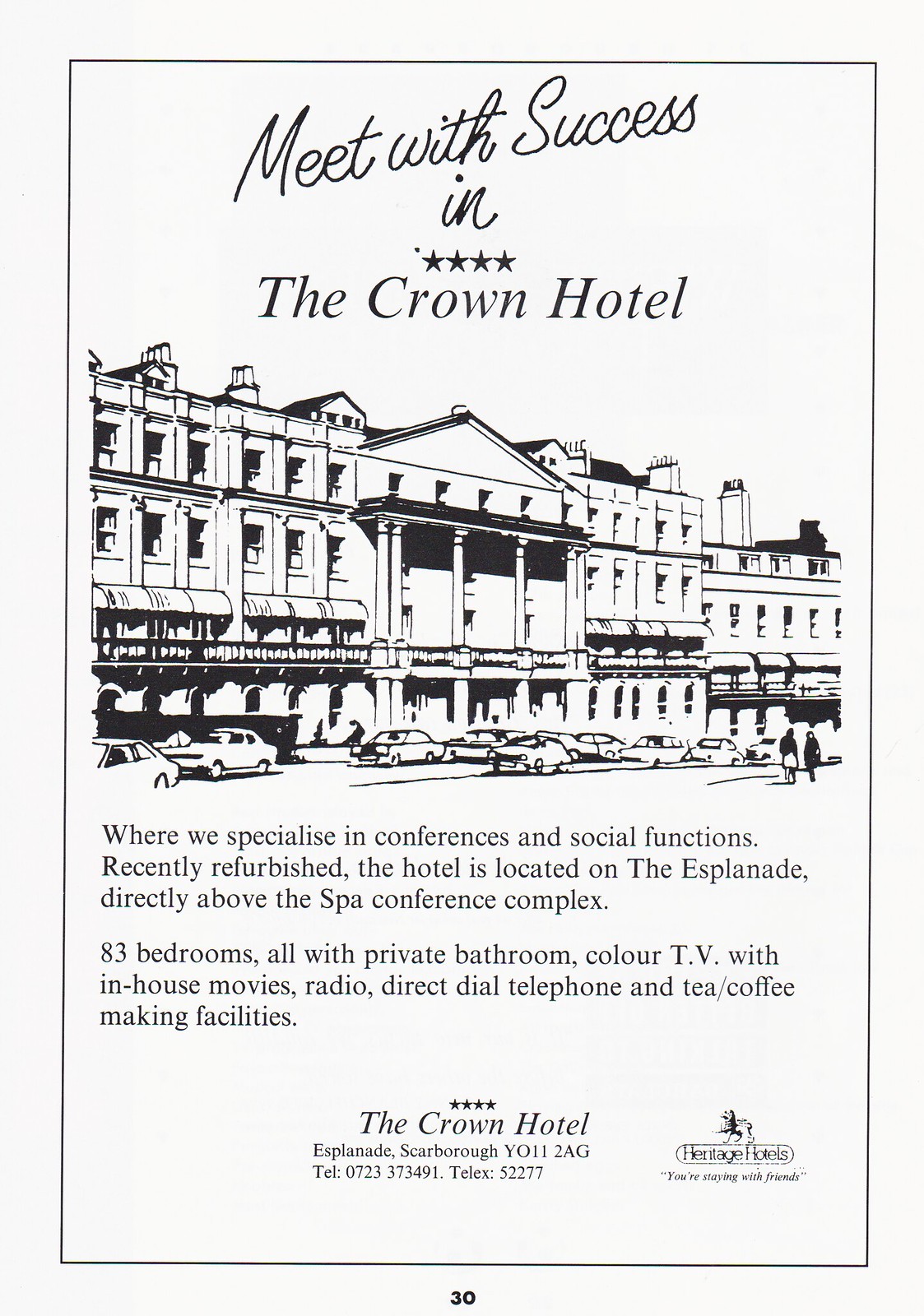This vertical, black-and-white advertisement resembles an aged, classic poster or card that promotes The Crown Hotel. Framed by a thin black border, the top of the image features the phrase "Meet with Success in" elegantly written in cursive, followed by four stars and then "The Crown Hotel" in bold print. Below this text is a detailed, somewhat cartoonish illustration of the three-story Crown Hotel, distinguished by prominent pillars at its entrance and numerous vintage cars parked in front, contributing to its old-fashioned charm.

Underneath the image, detailed information about the hotel is provided, highlighting its specialization in conferences and social functions. It notes that the hotel has been recently refurbished and is advantageously situated on the esplanade, directly above a spa conference complex. The advertisement makes a point of the hotel's 83 bedrooms, each equipped with private bathrooms, color TVs with in-house movies, radios, direct-dial telephones, and tea/coffee making facilities.

At the bottom, the address and contact number for The Crown Hotel are listed, reinforcing the nostalgic feel of the advertisement by emphasizing features like color TV as notable amenities. The overall design and text give the impression of a historical, reputable establishment perfect for business and social gatherings.